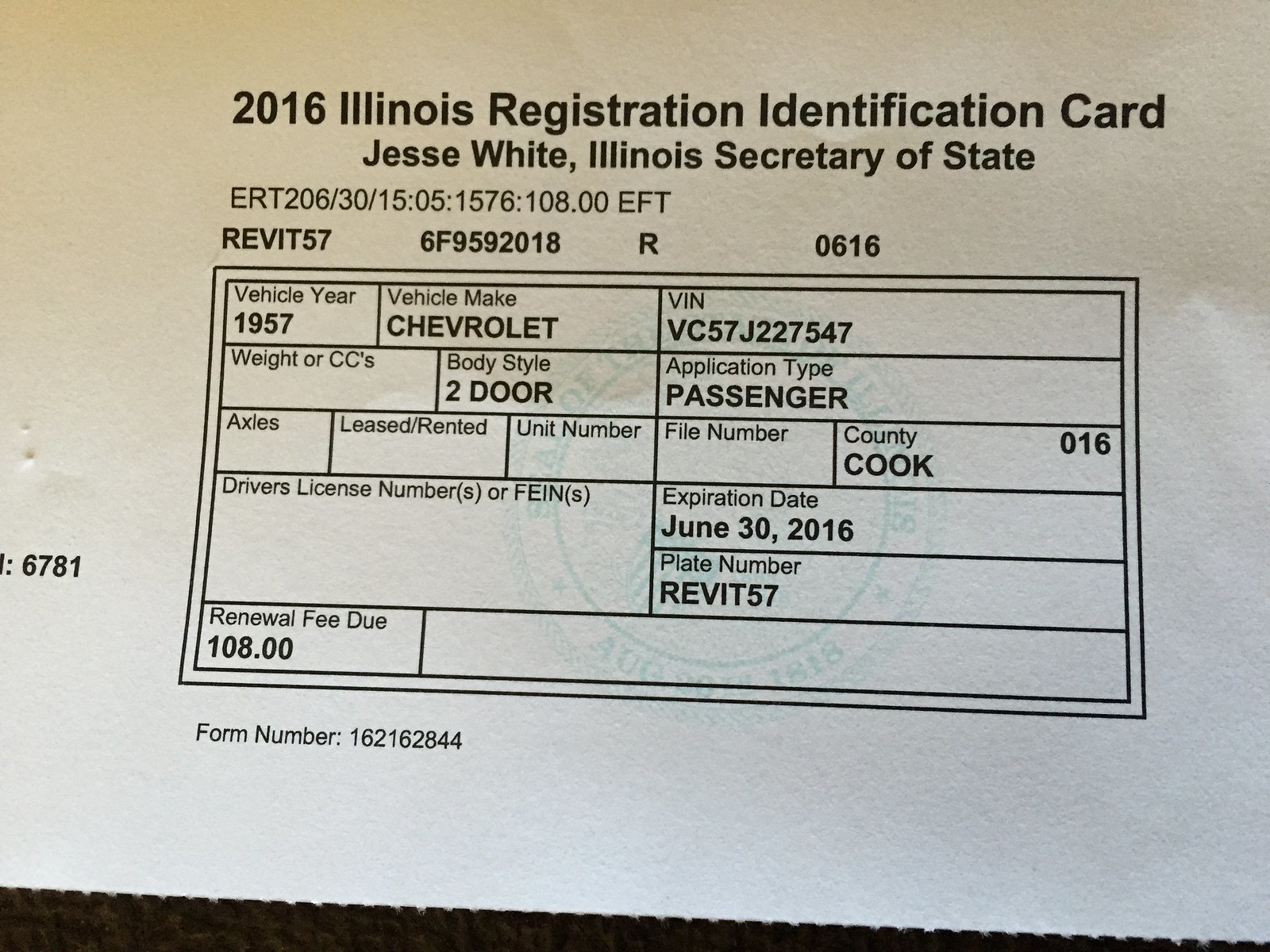A white sheet of paper with a slight gray shadow on it displays important registration information. At the top, black text reads "2016 Illinois Registration Identification Card, Jesse White, Illinois Secretary of State." Beneath it, in a lighter black font, is the code "ERT 206/30/15:05:1576:108.00 EFT." Following that, in a bolder black text, it states "REV IT576F9592018" and an "R" followed by "0616." Below, there is a double-outlined black square.

Further down, specific vehicle details are listed:
- Vehicle Year: 1957
- Vehicle Make: Chevrolet
- VIN Number: VC57J227547

Additional sections provide further details, though some are unfilled:
- Weight or CC: (empty)
- Body Style: 2-door
- Application Type: Passenger
- Axles: (empty)
- Leased/Rented: (empty)
- Unit Number: (empty)
- File Number: (empty)
- County: Cook (016)
- Driver License Numbers or FEINS: (empty)
- Expiration Date: June 30, 2016
- Plate Number: REV IT57
- Renewal Fee due: $108.00
- Form Number: 162162844
- Additionally, on the left side, the number 6781 is displayed.